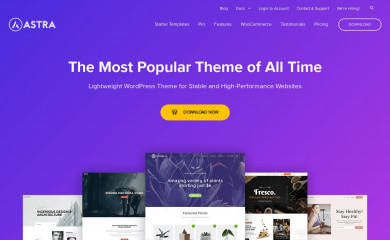This image is a digital advertisement for the Astra WordPress theme, prominently featuring a purple gradient background that transitions from a dark purple in the top left to a light purple in the bottom right. In the top left corner, there is a white logo consisting of the letter 'A' within a white circle, followed by the text "Astra" in white. Adjacent to this, there are several illegible website headings in white text. Centrally, the ad showcases the tagline "The most popular theme of all time" in large white text, with a subheading describing the theme as "fast, lightweight, and highly customizable." Below this description, there is a gold, pill-shaped button with black text that reads "Download Now," emphasizing a call to action. The lower part of the advertisement displays five example webpage layouts, each characterized by a darker top rectangle with illegible text and a white bottom rectangle featuring various images, collectively illustrating a diverse range of design possibilities.